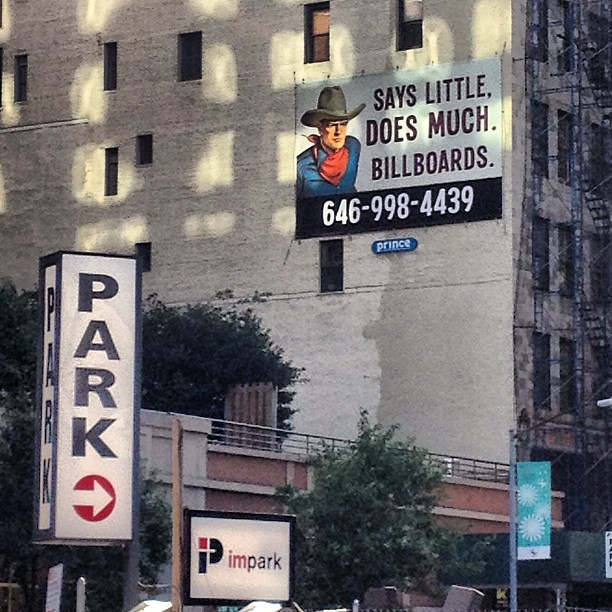A high-quality photograph captures a somewhat dilapidated tan building, featuring a mural of a cowboy wearing a tan hat, red bandana, and blue shirt. Above the mural, black text reads, "Little Does Much." Below this, a white phone number, 646-998-4439, is clearly displayed. Beneath the mural, a small white and blue sign reads "Prince." The building is adorned with black scaffolding and fire escapes. To the side of the building, a white sign with black lettering reads "Park," accompanied by a red and white directional arrow. Adjacent to it, a smaller black and red sign notes "I Am Park." The lower part of the building shows a brick structure, and a pole with a blue and white sign stands nearby.